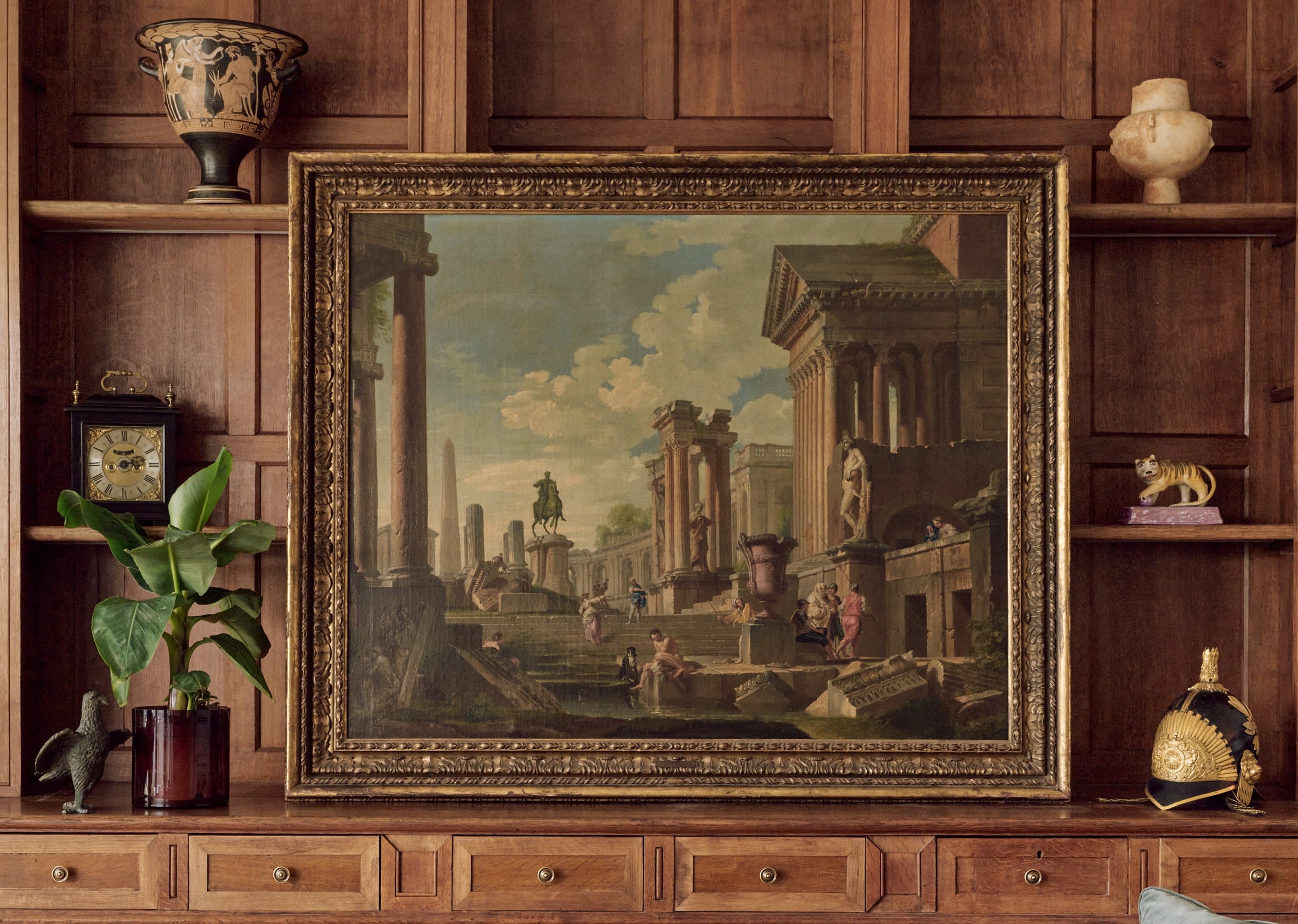The photograph features a detailed wood hutch mounted on a wall. The hutch has a series of six small tan and walnut colored drawers with handles, running horizontally along the bottom. The base of the hutch above these drawers is a solid plank of wood. On the left, a burgundy glass vase holds a tall green plant, while on the right, there's a gourd-shaped ewer or pitcher. Central to the image, leaning against the back of the hutch, is an ornate, gold-brown framed painting depicting an ancient city—possibly Roman or Greek—with stone columns and buildings in shades of tan and light brown. The scene includes a canal running through the middle, with a muted green sky and heavy graying clouds in the background. Above the painting, the hutch features additional cubes and shelves. On the upper left, there is a wood-framed, older-looking clock, and just below it, a small bird statue. On the top right shelf sits a rounded pitcher, narrower at the top and bottom, and beneath it a small yellow statue on a marble-like base. Other elements include a black helmet with gold detailing on the lower right, a decorative goblet-shaped vase on the left, and a small tiger statuette that looks like the base of a lamp.